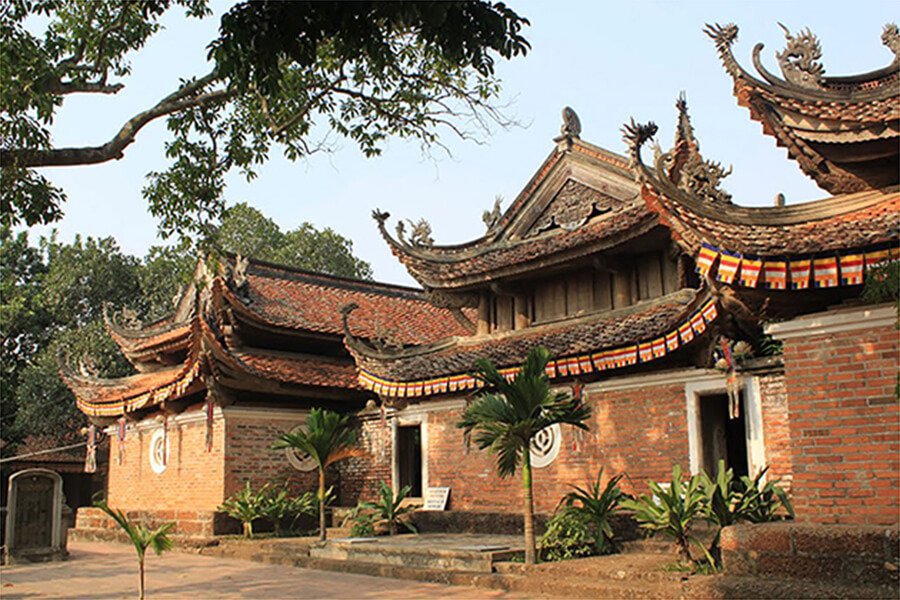This photograph showcases a trio of adjacent Chinese temples with distinct architectural elements. The temples, constructed with red bricks exhibiting various shades of red, feature pagoda-style, conical roofs adorned with intricate orange facades and terracotta clay shingles. The roofs are ornately decorated with figurines of dragons and mastheads, their corners curving elegantly upwards, emphasizing the classic Asian design. The central temple stands out with a prominent triangular tower topped by a figurine.

The image captures three such temples, although one appears only partially visible. The temples have multiple entrances and circular windows, creating a symmetrical and appealing facade. Each structure is accessed by a series of stairs, flanked by small shrubs and palm trees that add a touch of greenery. There is a plaque set in a cement pillar in front of the temples, though its inscription is not legible.

Surrounding the temples, lush green vegetation, including palm trees and overhanging branches, creates a serene backdrop. The left side of the photograph features additional tree branches, and beyond the buildings lies an empty ground. The sky above is clear and blue, providing a vivid contrast to the intricate and colorful temple exteriors.